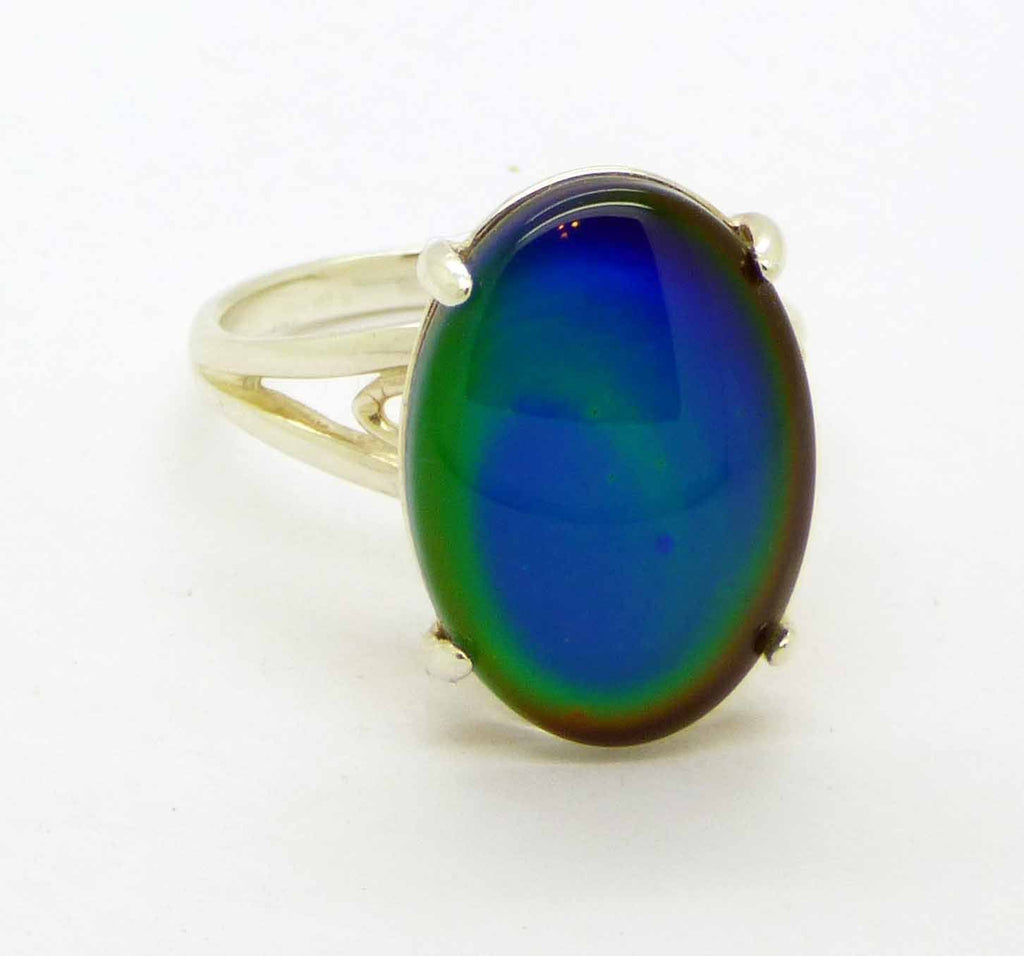This image features a unique, vintage-looking ring set against a completely white background, making the intricate details of the ring stand out prominently. The focal point of the ring is a large, highly polished oval cabochon stone, displaying a mesmerizing array of colors. The center of the stone glows with a radiant, royal blue hue, which gradually transitions to shades of green and brown, possibly resembling the look of a mood ring with its color-changing properties. The stone is securely held in place by four silver clasps. The ring itself has a simple yet elegant design, crafted from silver that forms a two-layered band joining into a single layer at the back. The overall impression is one of a substantial piece of jewelry, potentially covering a significant portion of the finger. This close-up photograph captures the exquisite beauty and detailed craftsmanship of the ring, making it a striking piece that stands out in any collection.